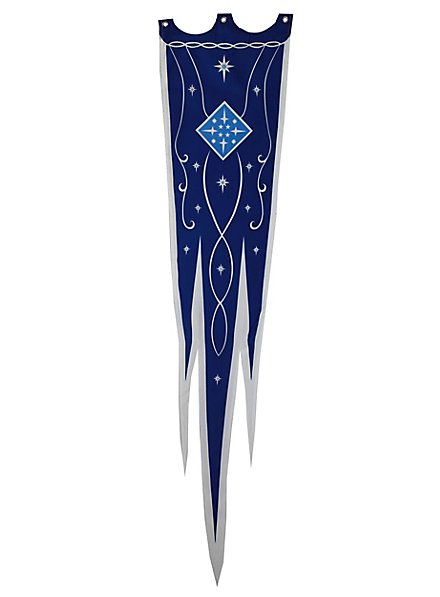The image depicts a distinctive banner or pennant flag, notable for its three pointed ends where the central point is longer than the ones on either side, giving it an arrow-like shape. The main body of the banner is dark navy blue with a detailed and ornate design. Central to the design is a light blue diamond or rhombus shape that features small white crosses, stars, and dots. Additionally, the banner is highlighted with a silver or gray outline, indicating it may have been hand-drawn or painted. The banner’s flat side is characterized by a scalloped edge with two inlets. Its overall decorative patterns give a sense of complexity and elegance, but without any text, the purpose or symbolism of the banner remains unclear.